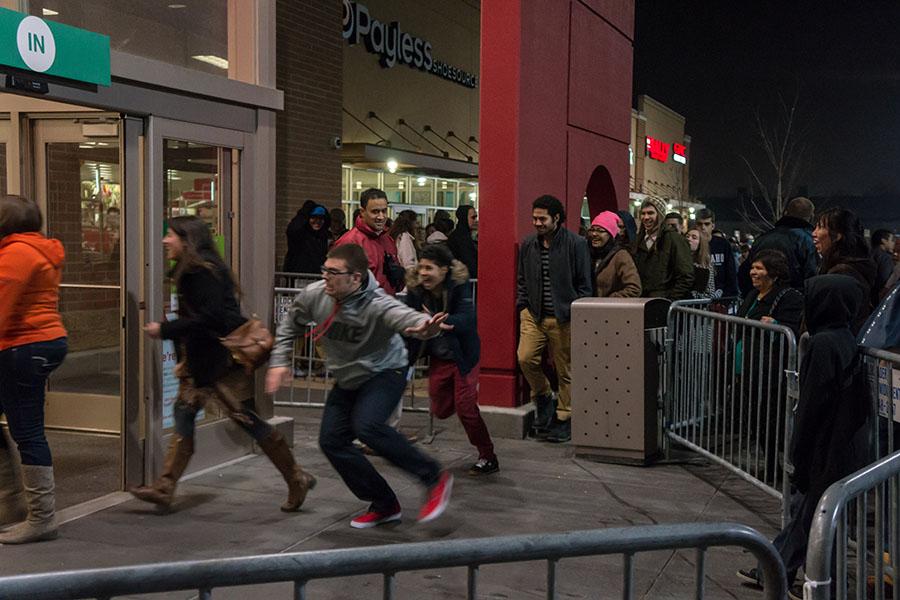The photograph captures a bustling nighttime scene of a large crowd gathered outside a store entrance, likely during a significant sales event such as Black Friday. The atmosphere is energized, with people dressed in warm winter clothing, eagerly rushing past metal barriers towards the store. The store entrance features a distinctive sign with "IN" written in green text inside a white circle. The central figure is a man with glasses, wearing a gray hoodie, jeans, and red sneakers, sprinting alongside others into the well-lit store. Surrounding him are several other excited individuals: a woman in an orange jacket with boots and jeans, another in a black jacket, jeans, and boots, and a third with olive skin in a blue jacket, red pants, and black trainers. In the background, you can catch a glimpse of Payless Shoes, hinting at the shopping center's layout. Laughter and smiles from the crowd convey the thrill and anticipation of securing irresistible deals.